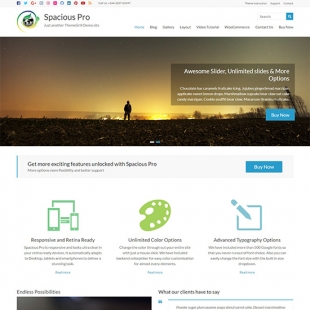This image showcases a vibrant promotion for "Texas Spacious Pro," a versatile technology platform. Various social media icons such as Facebook, Twitter, and Google+ are prominently displayed. 

The background features a bright sun shining over a landscape where a person is standing on dirt. The centerpiece of the display includes an appealing slider with unlimited slides and customization options. It promotes Texas Spacious Pro as a comprehensive solution, offering features like text layout, blog integration, video tutorials, and seamless contact options. 

A call to action encourages users to "Buy Now" to access more exciting features. The technological edge is highlighted by the presence of a smartphone and a computer monitor, both shown being responsive and fully functional. 

In the middle of the image, it touts unlimited color options with a color palette icon, advanced customization capabilities, appropriately designed options, and endless possibilities for users. 

The testimonial section is marked by a blue line followed by black text, set against a clean, white background. The promotion is rounded off with the website URL, www.texas.gov.